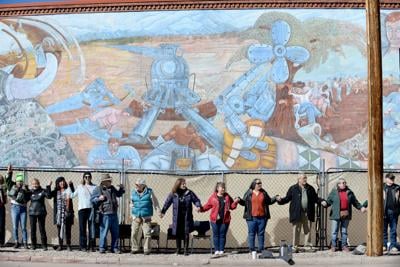A large group of people, comprising both men and women dressed in jeans and heavy jackets, stand in a line on a street, holding hands and forming a human chain. They appear older and seem united in solidarity, possibly as part of a protest. In front of them are bags and chairs, indicating they might have been there for an extended period. The group is positioned outside a metal fence and an electrical pole is visible off to the right. Behind the fence, a large, faded mural adorns the wall, displaying earthy tones of grays and browns. The mural features a collage of imagery, including what appears to be a blue structure at the center with beams emanating from it, suggesting a futuristic scene or a spaceship. The mural's muted colors create a somber backdrop for the determined gathering standing before it.